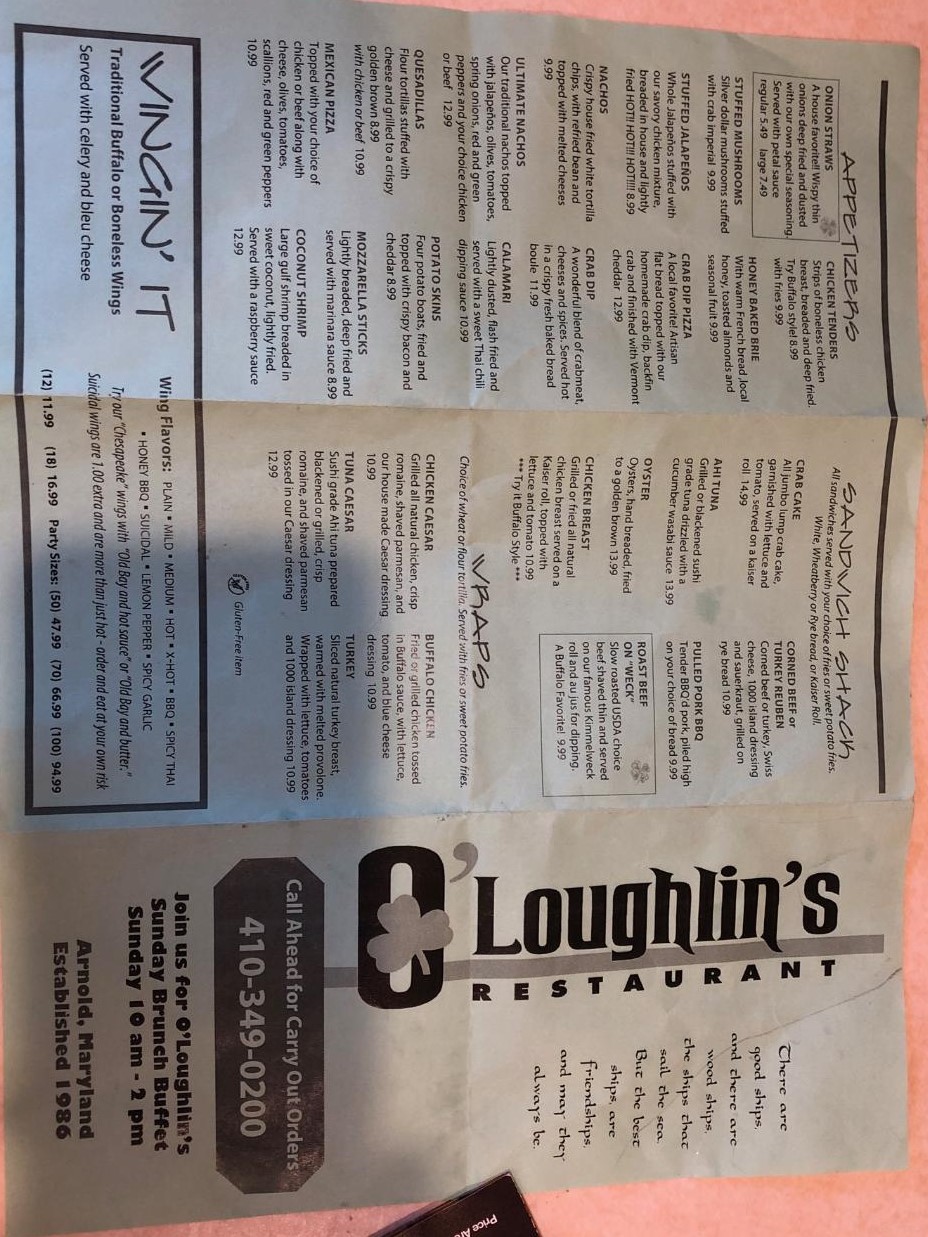Front page of the menu for Olo Lin's Restaurant, established in 1986 and located in Arnold, Maryland. The header prominently displays the restaurant's name and encourages customers to call ahead for carry-out orders at 410-349-0200. It also invites patrons to join their Sunday brunch buffet from 10 a.m. to 2 p.m. The menu items are arranged to the left of the header, including sections for appetizers, sandwich shacks, and wraps. At the bottom left corner of the menu, there's a section called "Winging It," featuring traditional buffalo or boneless wings served with celery and blue cheese.